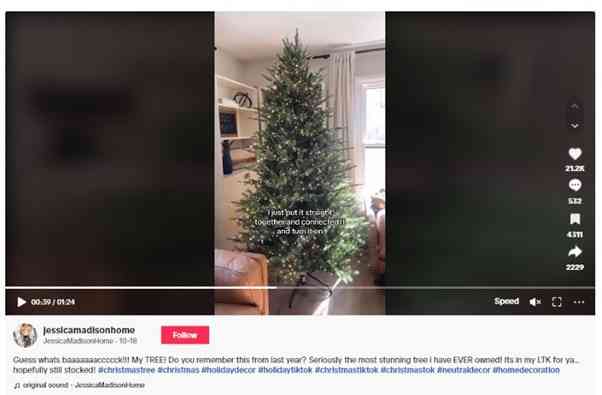In this image, we see a screenshot of a video playing on a sensor screen. The video itself features a festive scene with a Christmas tree prominently displayed in the center. The tree is green with some darker highlights and is situated on the floor of a room. This room has white walls and a white ceiling, contributing to a bright atmosphere. Behind the tree, slightly to the right, is a window covered by a white curtain that is connected to a black rod at the top. Light streams softly through the curtain, illuminating the scene.

To the right of the Christmas tree stands a white cabinet, while a cozy brown couch is positioned in the bottom left corner of the room. A white play mat or rug is also visible in this corner, adding to the room's decor.

The sides of the video frame, including both the left and right edges, are dark and blurry, suggesting a sense of focus on the central scene. On-screen video controls are visible, with a play button and a timestamp located at the bottom left corner. The bottom right corner hosts icons for speed adjustment, mute, maximize, and options.

To the right of the video, there are additional icons for liking, commenting, marking as a favorite, and sharing the video. Below the video, the channel name "Jessica Madison Homer" can be seen, accompanied by a red subscribe button. Underneath this button, the channel description is present though the text is grainy and hard to read. Hashtags are written in blue, while the channel description is in black. Despite the graininess of the image, the festive spirit of the scene is clearly conveyed.